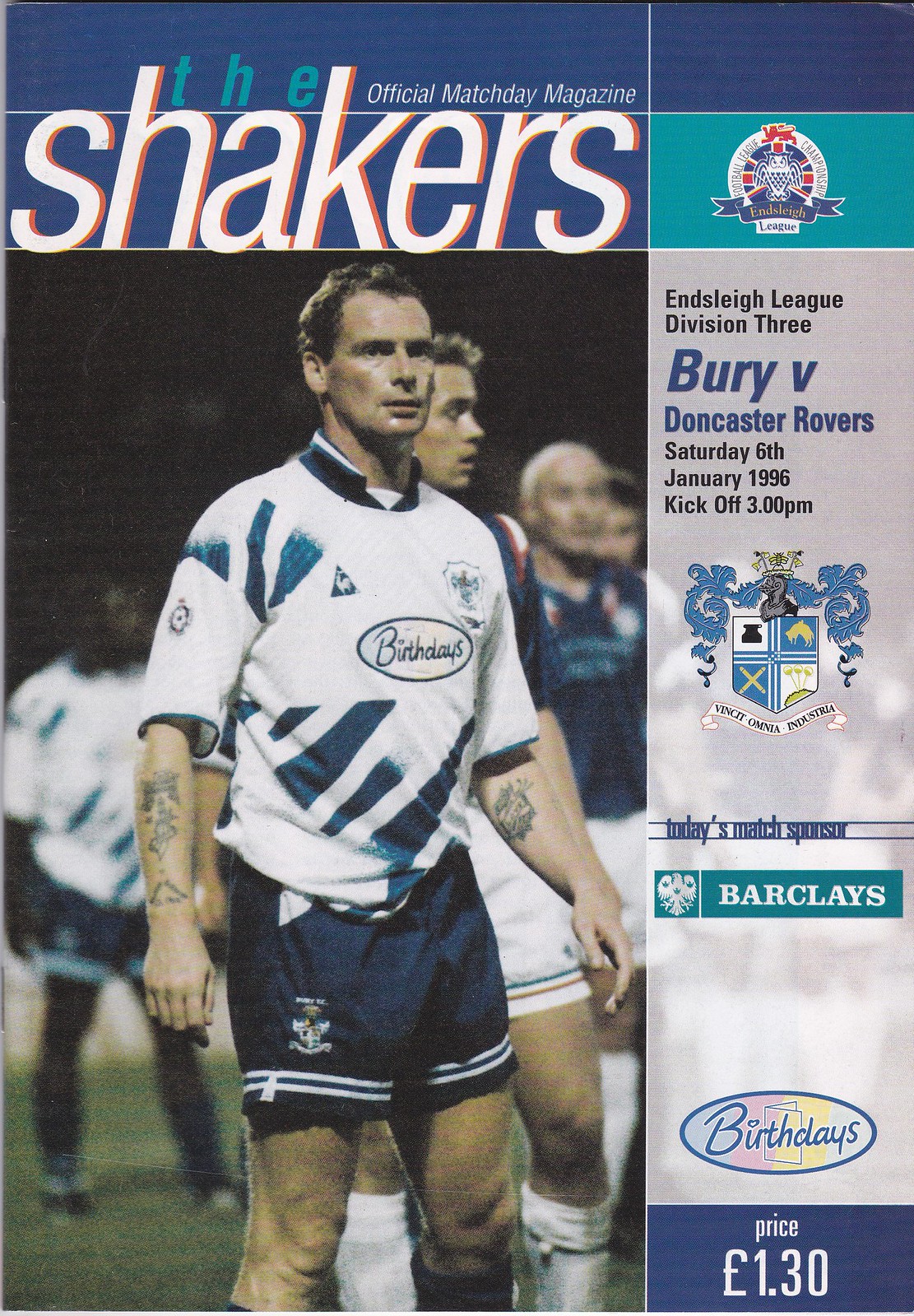This tall rectangular image appears to be the front page of an old sports program or magazine advertising a soccer match. At the top, there is a dark blue bar with turquoise letters spelling "the," followed by "Official Match Day Magazine" in small white letters. To the right, in much larger white letters with an orange shadow, it reads "Shakers." Adjacent to it, in a lighter blue to turquoise rectangle, there is a symbol featuring an owl with spread wings, along with the text "ENSLING LEAGUE." 

Dominating the left side and extending downwards is a photograph of a soccer player in a white and turquoise jersey, presumably the team captain, with several players visible behind him, suggesting he is part of a team lineup. The image gives an old-time feel, indicated by the faded appearance and the dated style of clothing.

Below, a semi-transparent gray bar stretches almost to the bottom, detailing "ENSLING LEAGUE Division Three BURY V DONCASTER ROVERS Saturday 6th January 1996 kickoff 3 p.m." Underneath, a shield crest is divided into four sections – a black anvil, crossed swords pointing downward, a tent, and a bunch of flowers. Further down, it mentions "today's match sponsor" with a bird adorned with three small hearts labeled "Barclays" and "birthdays." The bottom right corner lists the price as "1.3 euros."